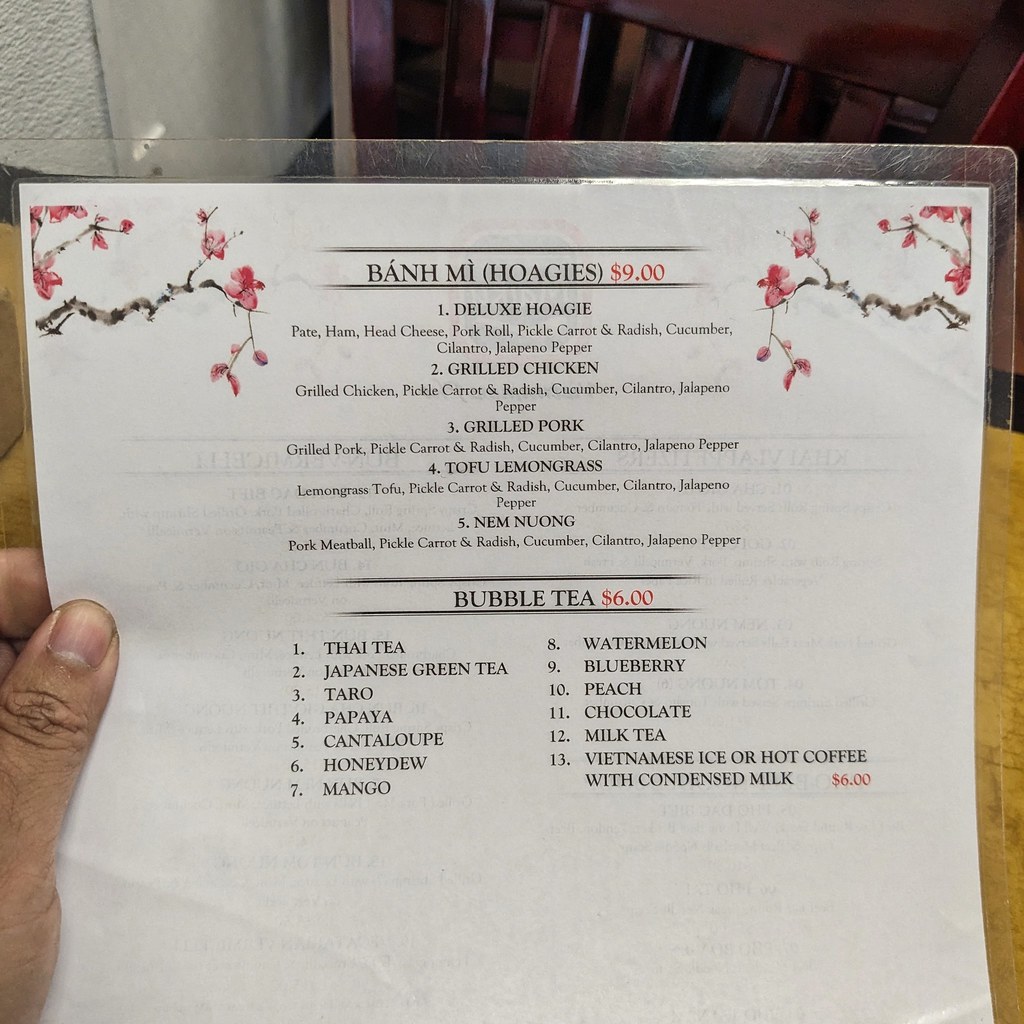The photograph captures a detailed scene at a restaurant, featuring a close-up of a menu held by a left hand with brown skin. The human hand firmly grasps the white menu, with the thumb holding the front and fingers supporting the back. The background showcases a yellow table and an empty, dark brown chair, adding depth to the setting. To the left, a wall is visible, alongside faint shapes indicating another table, further suggesting the restaurant environment.

The menu itself is adorned with artistic branches in the top left and right corners, embellished with pink flowers. It presents a variety of items, with the first listed item being “banh mi – hoagie,” hinting at a diverse linguistic influence. The menu details five different hoagies, each priced at $9, including options like deluxe hoagie, grilled chicken, grilled pork, tofu, lemongrass, and nam nuong. Below, a category dedicated to bubble tea lists 13 flavors such as Thai tea, Japanese green tea, taro, papaya, cantaloupe, honeydew, mango, watermelon, blueberry, peach, and chocolate, all priced at $6 each. Additionally, Vietnamese iced or hot coffee with condensed milk is offered. The artistic design, varied menu, and detailed setting contribute to the lively atmosphere of the scene.